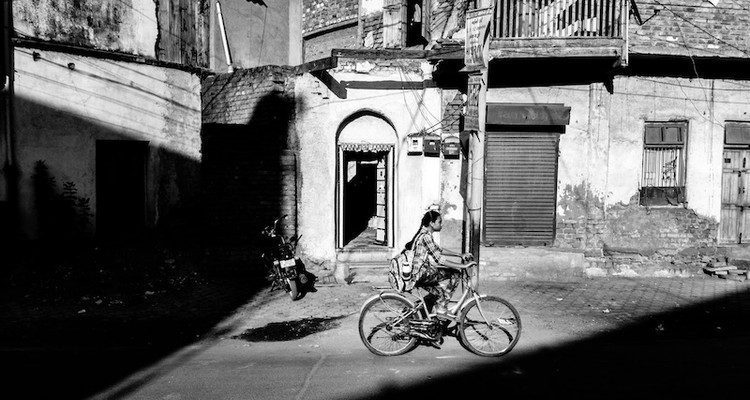This black and white photo captures an evocative scene set in a foreign locale, distinctively not in the United States. In the middle of a dilapidated courtyard stands a young girl on a full-sized bicycle, her long dark hair styled into a single braid trailing down her back. She wears a long-sleeved plaid shirt, rolled up to her elbows, and dark pants, suggesting a casual and practical outfit possibly adorned with a large backpack extending low on her back. 

The courtyard and surrounding environment tell a vivid story of age and decay. The ground appears dirty, possibly cobblestoned. The building to the right of the image displays a closed corrugated metal garage door, flanked by two windows, with an old arched door nearby—a motorcycle parked in front of it adds to the scene’s texture. Above, a wooden balcony seems rickety and broken windows hint at long-term neglect. 

To the left, darker, shadowed structures further emphasize the decay with wooden siding falling off and an awning hanging unevenly. An open doorway with a partial curtain adds an almost ghostly presence to the otherwise desolate environment. Ambient shadows suggest the photo was taken early in the morning or late in the day, with low-angle sunlight providing half-shadow across the courtyard, bathing the girl in full sunlight. The overall setting is somber and atmospheric, replete with a sense of timeless, poignant history.